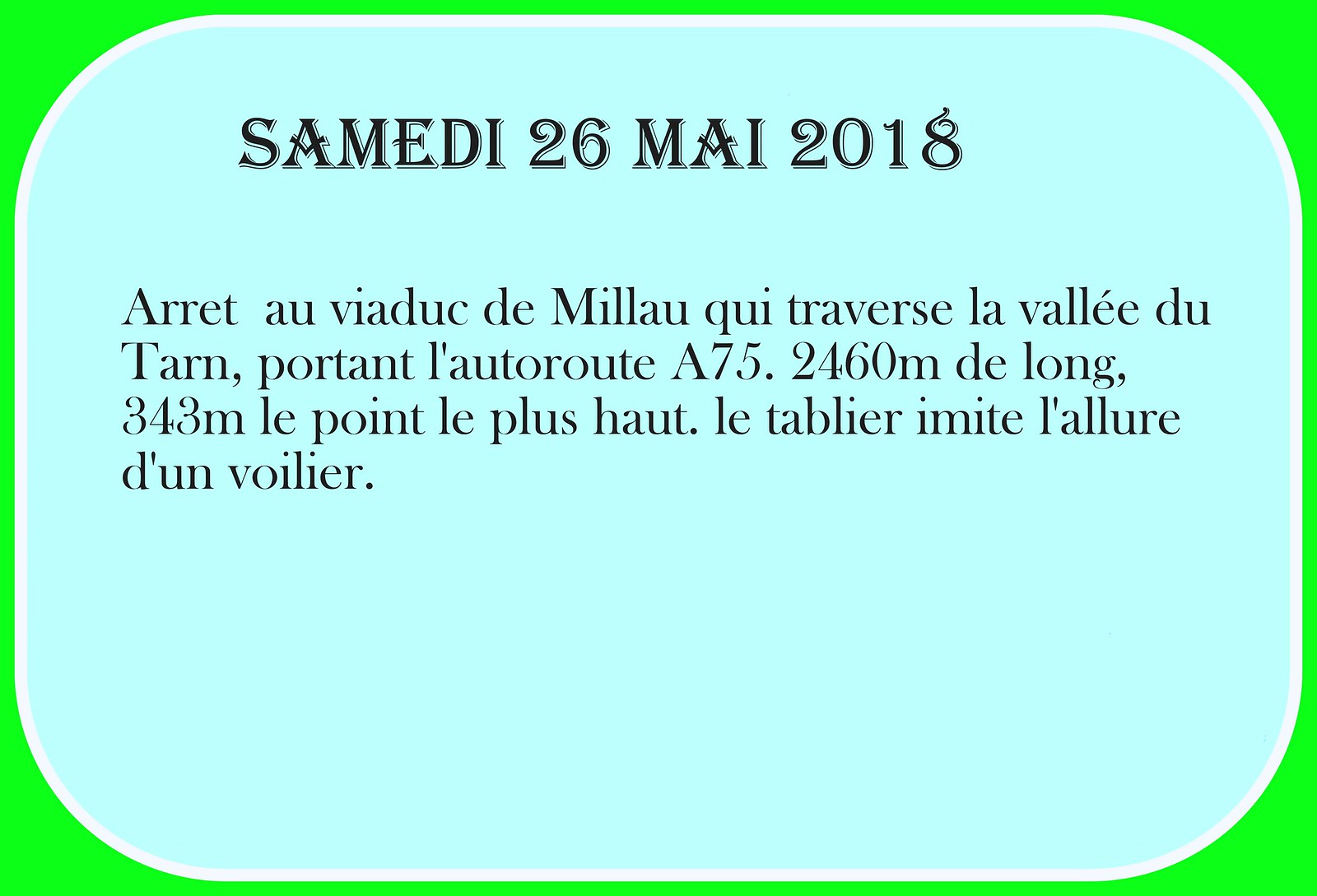The image depicts a sign with a striking background of bright greens, nearing neon but not quite reaching that intensity. This vibrant backdrop frames a large central rectangle that almost fills the entire sign, featuring a light blue, nearly turquoise backdrop. The main title on the sign is printed in bold black letters, reading "SAMEDI 26 MAI 2018." Below this title, in smaller black print, the text continues in French, stating: "Arrête au viaduc de Millau qui traverse la vallée du Tarn portant l'autoroute A75. 2460 m de long, 343 m le point le plus haut. Le tablier imite la lueur d'une voie lactée." This roughly translates to "Stop at the Millau Viaduct which crosses the Tarn Valley carrying the A75 motorway. 2460 meters long, 343 meters at its highest point. The deck imitates the glow of the Milky Way." The design includes a white outline around the light blue section, providing a finished and clean look to the informative sign.